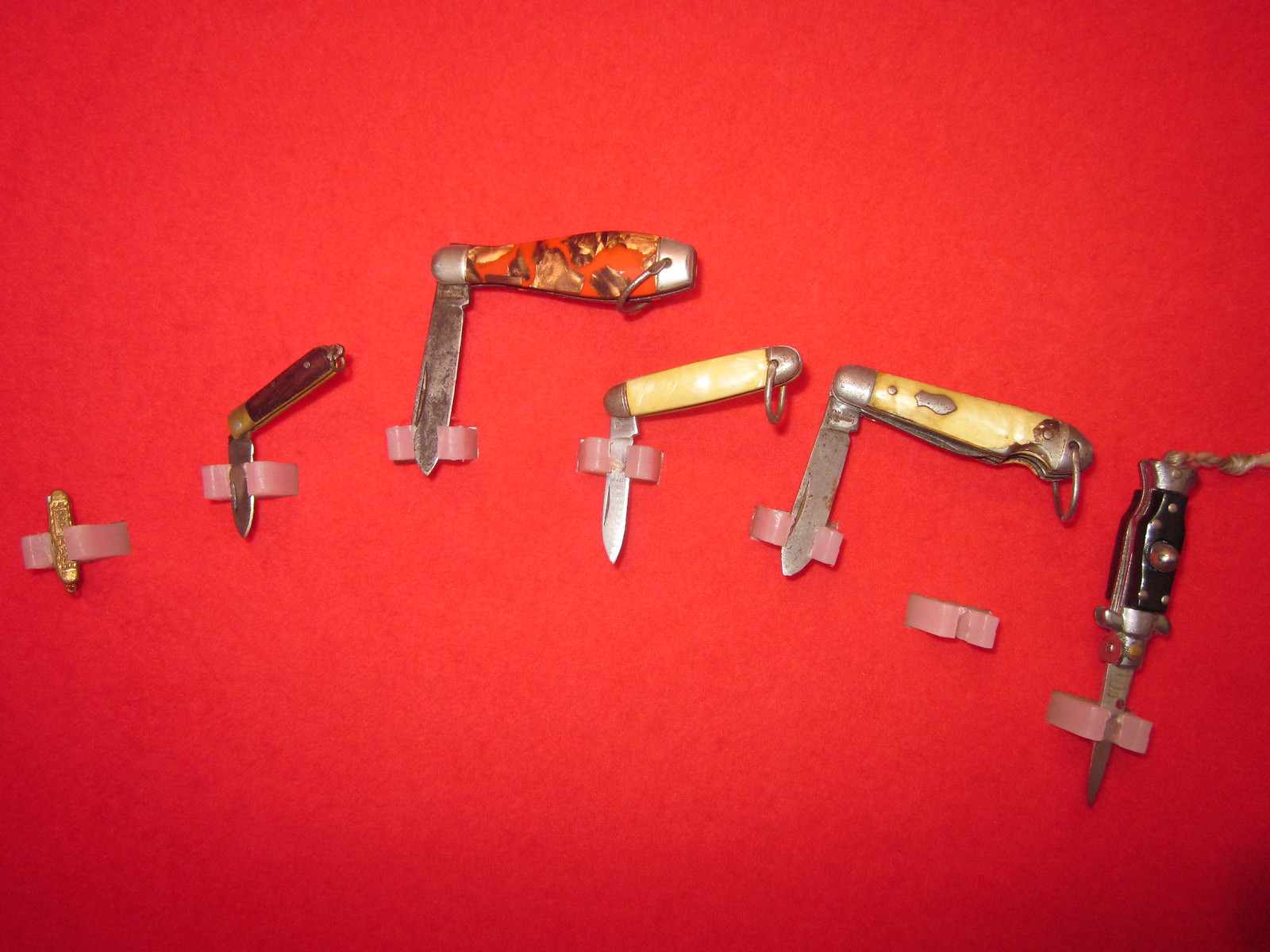In this image, six pocket knives are meticulously arranged on display against a red wall or table surface. Each knife is secured in place by small, white plastic clips that grip the blades, with the handles left free. The knives vary in color and design, contributing to a rich, intricate composition. There is one black-handled knife that is fully extended, prominently positioned at the far left. Adjacent to it is a yellow-handled knife with its large blade partially folded out. Another smaller yellow-handled knife shows a similar partially extended blade. A red and gold-handled knife, also partially open, sits nearby. Additionally, there is a small dark wooden-handled knife, and beside it, a tiny golden knife with its blade fully closed. These knives appear aged with some showing signs of wear, imparting an antique feel to the display. Notably, an unused seventh mount suggests space for one more knife, adding an element of incompleteness to the otherwise detailed and carefully curated arrangement.